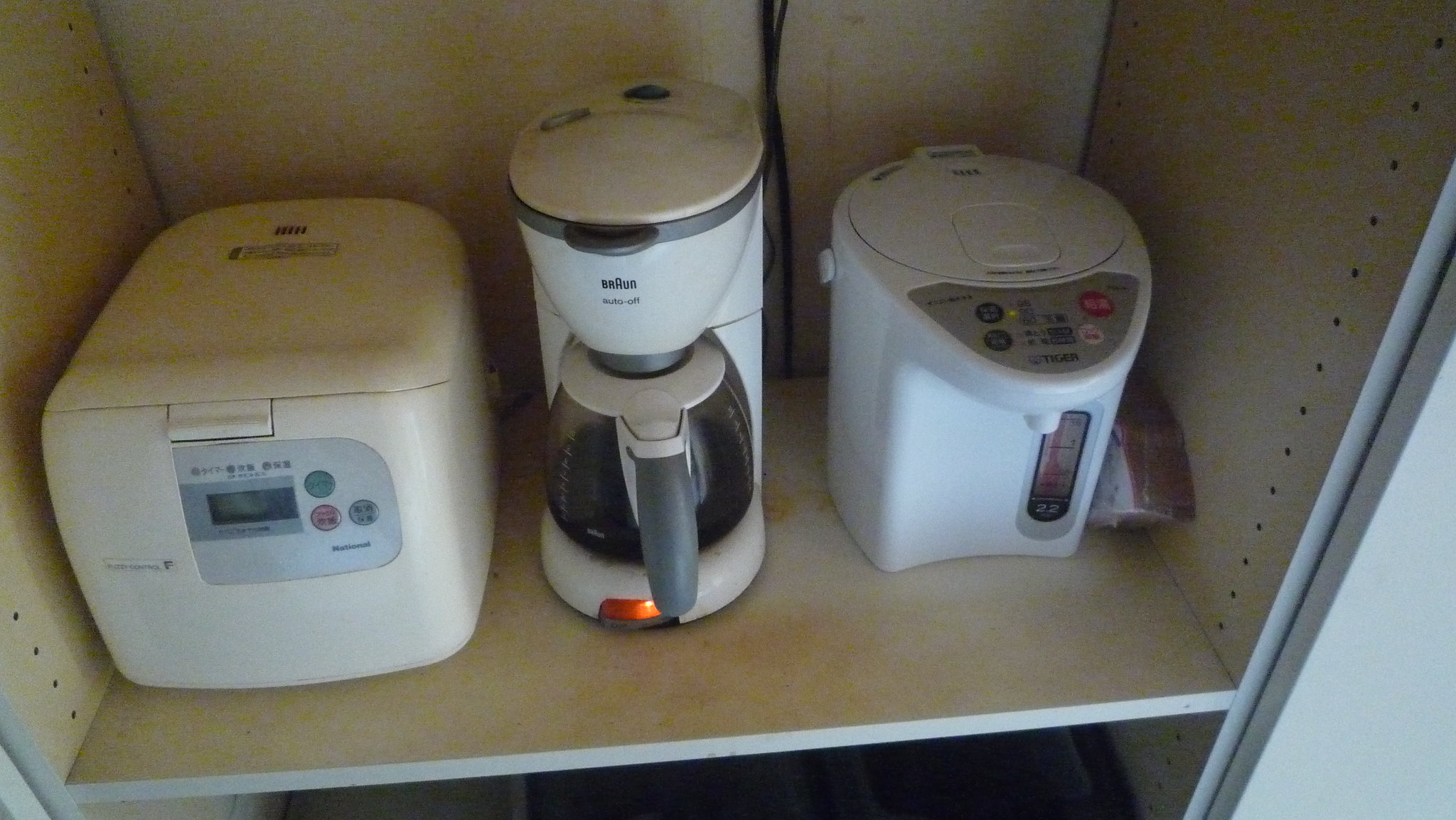The image showcases three white kitchen appliances arranged neatly on a beige-like shelf with light brown, tannish walls in the background. On the left, there is a cube-shaped device resembling either an oven or a rice cooker, identifiable by its three buttons in green, red, and blue, a small display window, and a top latch for opening. In the middle sits an electric coffee pot labeled 'Brawn' with an 'auto-off' feature. The gray-handled coffee pot is actively brewing, as indicated by an illuminated light and visible black coffee inside the pot. On the right, there's another white kitchen appliance featuring a gray bottom, a front display, and various buttons with unreadable lettering near the top. The white shelf holding these appliances has a whitish-gray outer ledge, enhancing the organized kitchen setting.